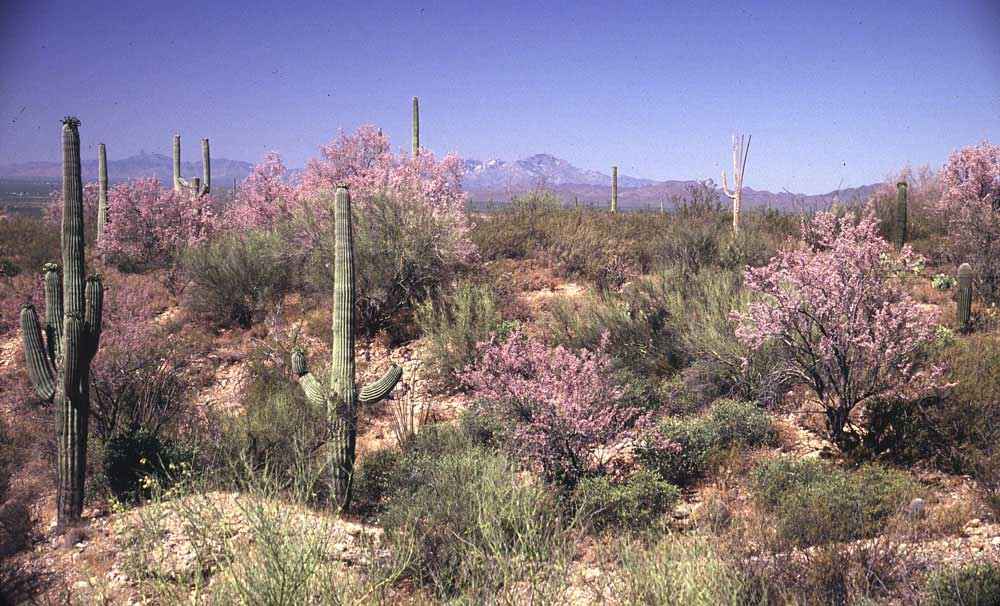The image depicts an outdoor desert scene, featuring a rich and wild landscape. The photograph, slightly aged with soft, washed-out colors and a hint of pixelation, captures a bustling desert environment that is far from barren. Dominating the scene are tall cacti with multiple arms in varying shades of green, set against uneven ground in the foreground with a boulder stretching across from left to right, characterized by its humped surface. Scattered throughout are different types of wild grasses in diverse green hues, dotted with brown patches. Among these grasses, bushes with pale pink flowers add bursts of color. Further back, the horizon displays a gently undulating mountain range. The sky above, mostly blue with a subtle purplish tint likely due to the photograph's age and quality, stretches across the top third of the image, lending a unique tone to the overall scene.